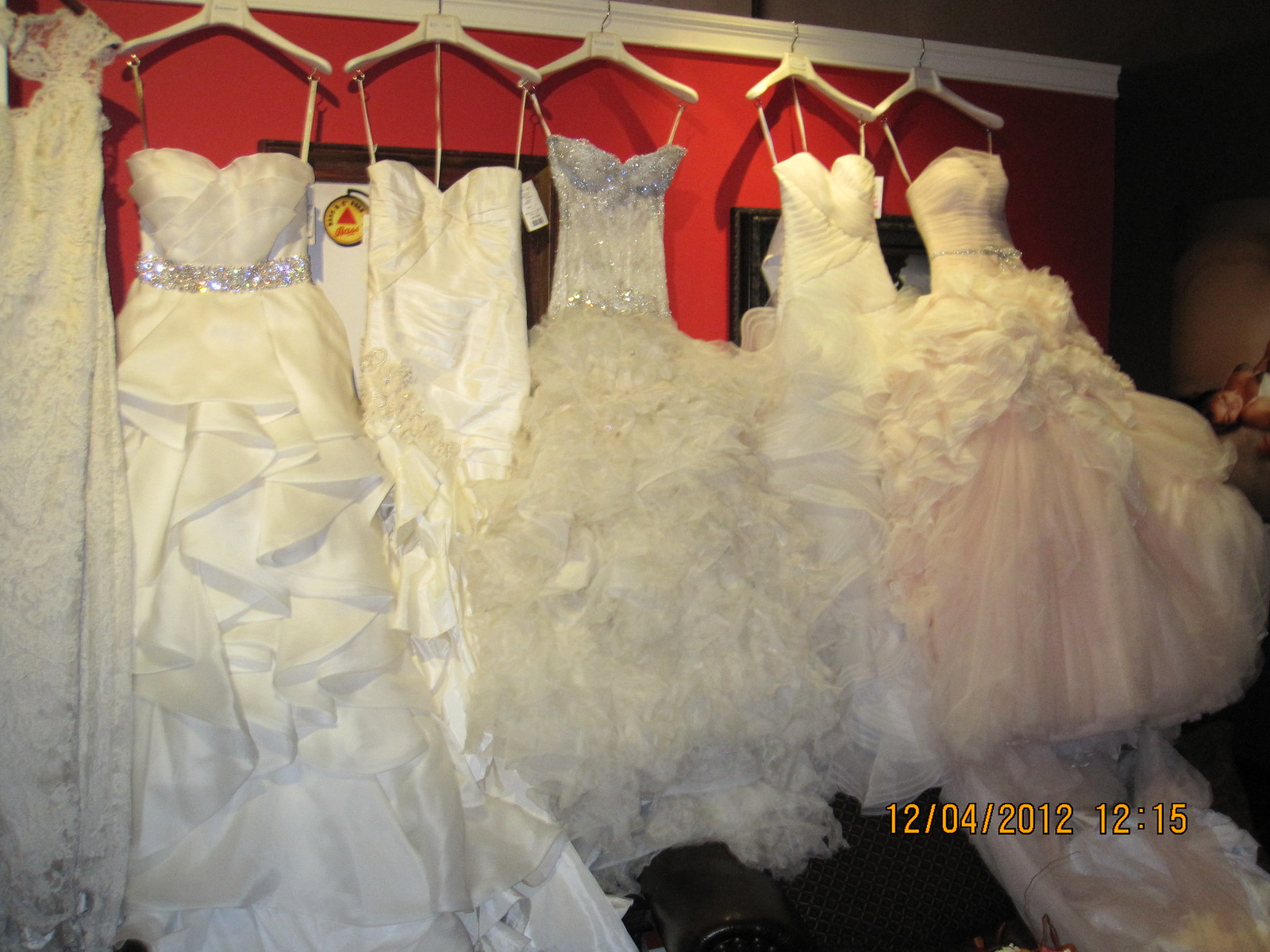This detailed photograph, likely taken with a flash on a digital camera, captures six luxurious wedding gowns hanging on white coat hangers against a striking red wall, dated December 4, 2012, at 12:15 AM or PM in orange text at the bottom right. The setting appears to be a store, evidenced by tags on some dresses and an illustration of a reclining woman visible on the far right. Each gown boasts a unique design with elements like strapless bodices, ruffled skirts, and materials ranging from taffeta to satin. Some dresses feature intricate silvery or diamante beads, especially one in the middle adorned with silver crustaceans and flurry-ish tassels with long pink trains. The hangers are mounted on a white hook rack, providing an orderly display amidst the vibrant red background, punctuated by small windows adding a touch of natural light to the scene.